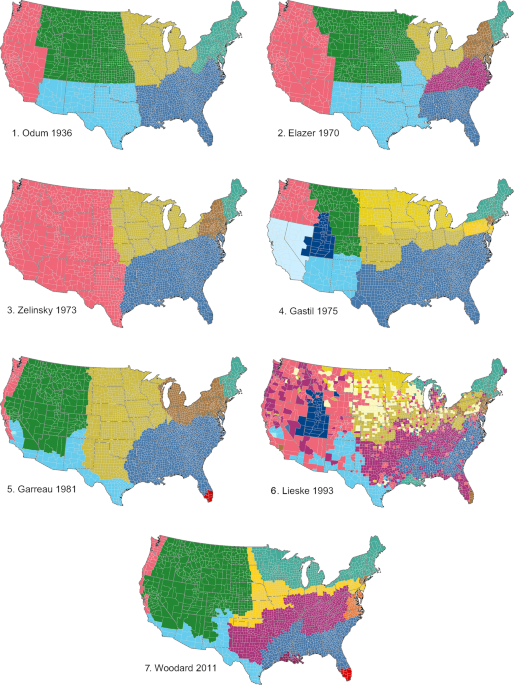This portrait-oriented image features seven colorized maps of the United States, each visually representing different regions with color blocks. The maps are arranged in two columns of three, with a seventh map centered below the bottom row. These maps are possibly depicting different periods in time and maybe related to voting or demographic changes. Each map is accompanied by a numbered label and a name with a date to the right. 

From the top left, the sequence is as follows:
1. Odum, 1936: Featuring divisions in pink, green, yellow, blue, and light blue.
2. Elazer, 1970: Displaying various regions in similar but more detailed color separations.
3. Zelensky, 1973.
4. Gastille, 1975.
5. Gouraud, 1981.
6. Lieske, 1993.
7. Woodard, 2011: Located at the bottom center, completing the lineup.

The text is black and placed to the left of each map. The colors used across the maps include pink, green, blue, yellow, purple, brown, and teal, with regions divided differently in each map, illustrating changes over time in a detailed and colored format.